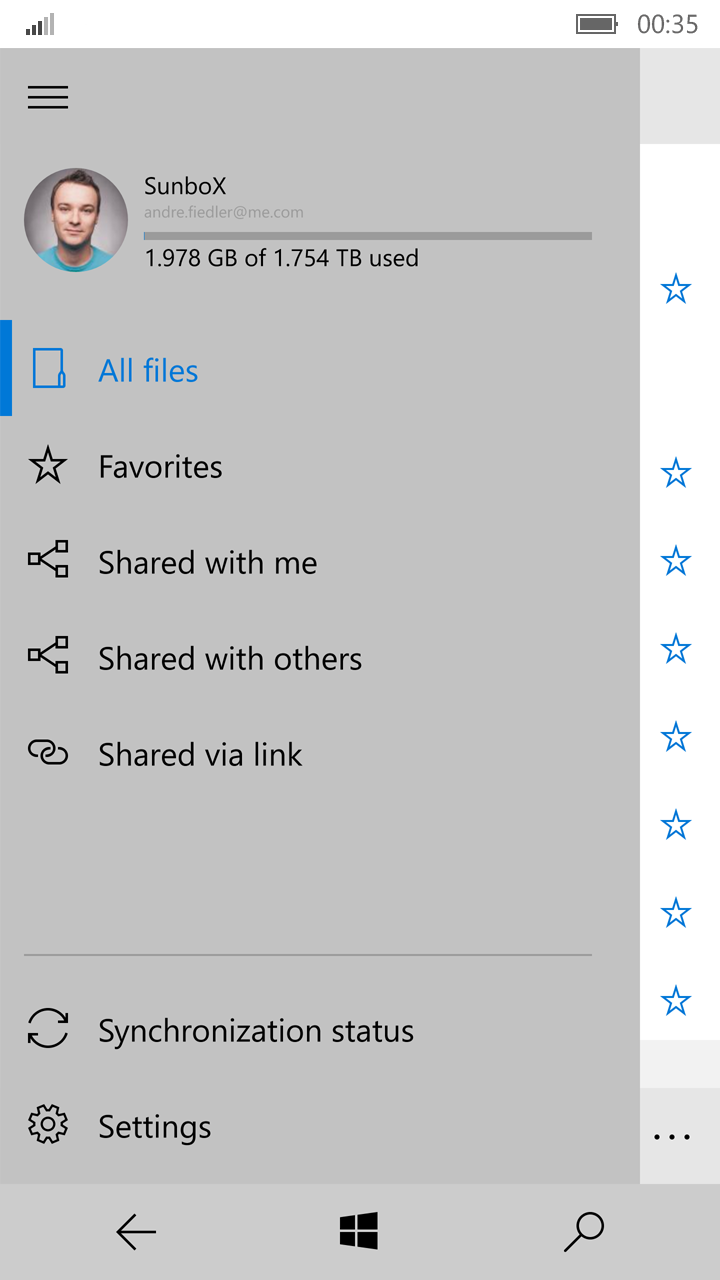The image is a mobile screenshot, likely from a Windows phone or displaying a Windows software interface. In the top left corner is a hamburger icon, presumably for accessing additional settings. Next to it, there is a profile picture of a clean-shaven white man with short brown hair, wearing a pale blue shirt. His eye color is not discernible. To the right of the profile picture, the text reads "Sunbox" and "Andre Fielder at me.com," indicating the user's Apple email address.

Below this header, storage usage information is displayed: 1.978 GB used out of a total 1.754 TB, indicating ample storage space available on the device. Beneath this, a series of icons and labels are listed:

1. A piece of paper and marker icon (highlighted in blue) labeled "All Files."
2. A star icon labeled "Favorites."
3. A typical share icon (a square with two lines extending from it) labeled "Shared with Me."
4. The same share icon labeled "Shared with Others."
5. Two link icons labeled "Shared by a Link."
6. Two arrows resembling a recycling symbol labeled "Synchronization Status."
7. A cogwheel icon labeled "Settings."

At the bottom of the screen, there is a left-pointing arrow, a Windows logo, and a magnifying glass icon. To the right are additional elements including eight outlined stars and sections indicating cellular reception (three out of five bars), a charged battery, and the time 12:35 AM.

Based on the screenshot, this appears to be a Microsoft Windows storage management interface.